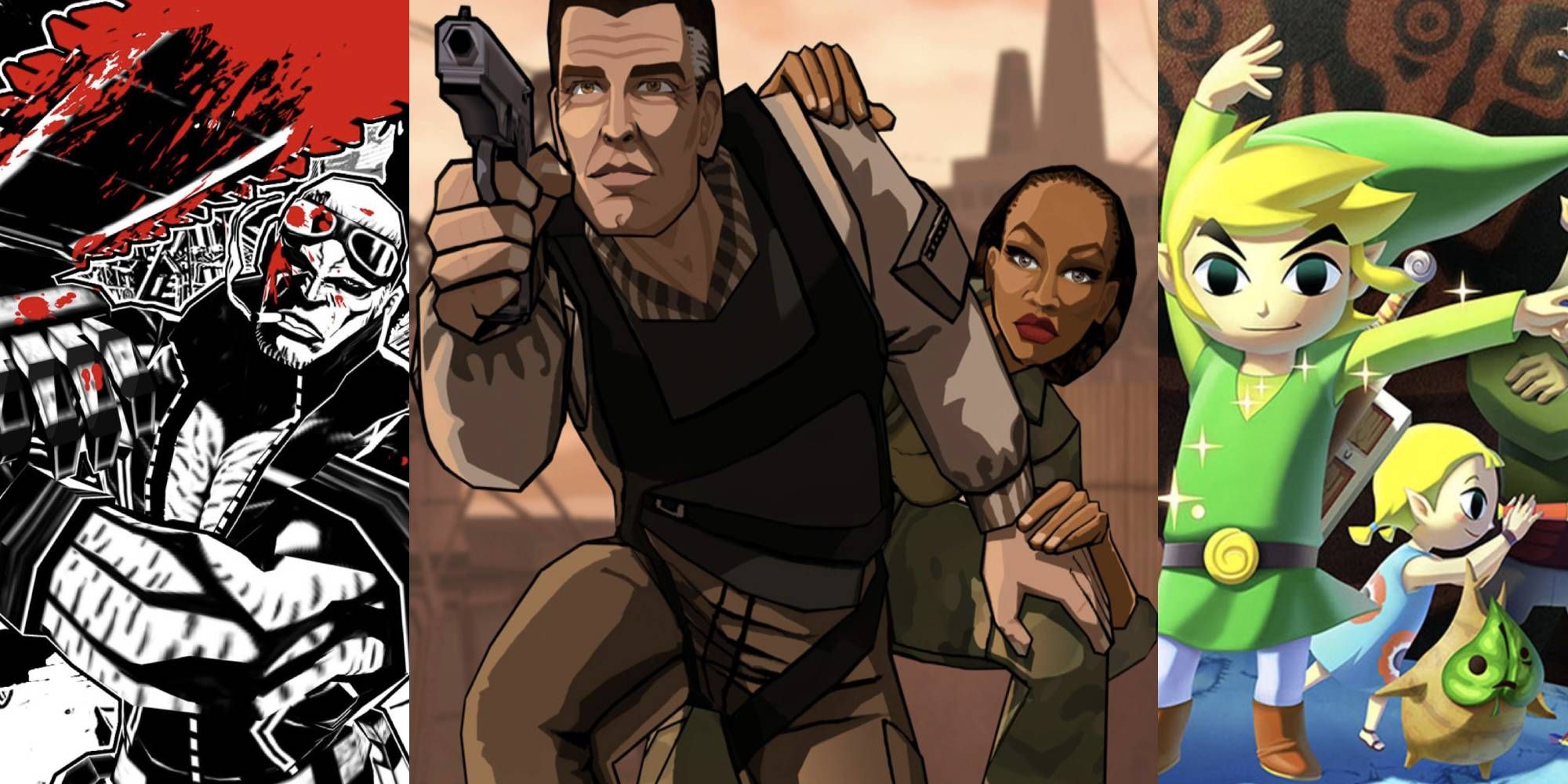The artwork comprises three distinct cartoon panels, each rendered in a unique style. The left panel features a steampunk-esque villain, drawn in pen and ink with a palette limited to black, white, and red. This menacing character, clad in black, sports red knuckles and facial marks, and is biting down on a cigarette with smoke curling from it. The sky above him is streaked with red, suggesting a scene of bloodshed. The central panel, depicted in black and sepia tones, showcases a tense moment: a man in a tactical suit is crouched and aiming a gun forward, while a woman, depicted with darker skin, clings to his shoulder, peering out anxiously from behind him as he shields her. Their dire situation is palpable, conveying a sense of danger and protection. The right panel shifts to a more whimsical tone, portraying a young blonde boy reminiscent of Peter Pan, dressed in traditional green attire with a pointed hat. Behind him stands a little girl, also with yellow hair, who peers through a spyglass towards the right, adding a sense of adventurous curiosity to the scene. Despite their differing styles and moods, the panels together create a rich tapestry of storytelling through visual art.